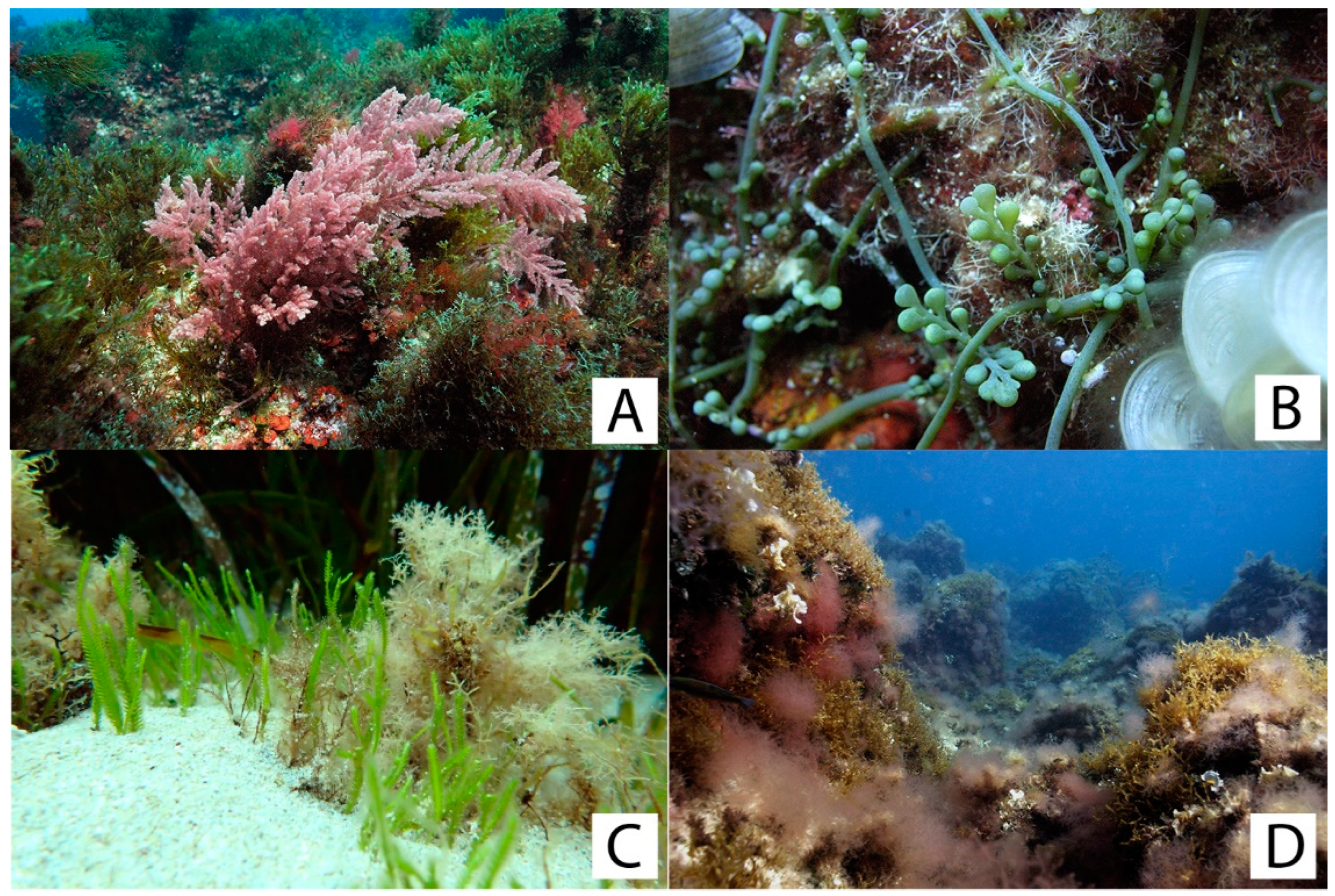This rectangular image, wider than it is tall, is divided into four sections, each marked in the bottom right corner with white squares containing black letters: A in the top left, B in the top right, C in the bottom left, and D in the bottom right. Each section features a different underwater scene. 

Photograph A showcases a vibrant pink sea anemone surrounded by green marine plants. Photograph B displays intricate details of underwater flora, resembling green grapes and seaweed with white circular elements scattered around. In Photograph C, seagrass extends from the ocean floor, accompanied by bluish coral and floating white seaweed, likely influenced by the camera's lighting. Photograph D presents an expansive view of the ocean floor, decorated with various intricate sea plants and ridges, highlighted by a white sea anemone in the foreground against a backdrop of dark green flora.